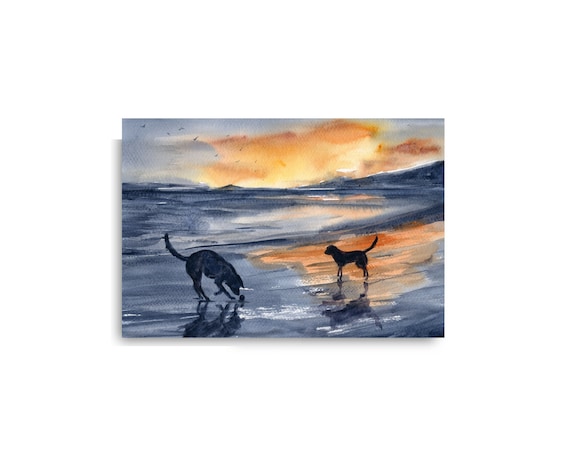The illustration depicts two dogs on a beach under a grey sky with patches of orange clouds likely from a sunset. The beach and the sea share a grey hue with hints of white, possibly reflecting the evening light. The painting captures the dogs facing each other, with their tails pointed in opposite directions. The dog on the left is sniffing a small ball-like object on the ground, while the dog on the right looks off to the left. In the distance, gentle waves roll in and faint outlines of seabirds can be seen flying in the sky. There's a small slope in the top right corner, adding subtle depth to the scene. The overall ambiance of the illustration is serene, with the reflective quality of the wet sand beneath the dogs suggesting the tide is coming in.